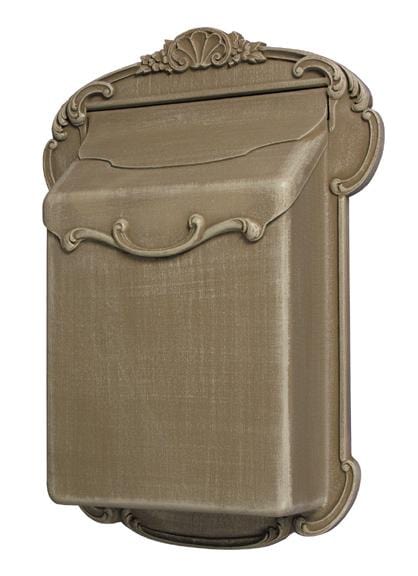The photograph showcases a vintage-style, wall-mounted mailbox set against a pristine white backdrop. At the center of the image, the mailbox, colored in a light tan or coppery brown, stands out with its ornate design and elegant curves. The mailbox elongates vertically more than horizontally, featuring a lift-top flap adorned with seashell-like textures and wavy designs. This flap, which includes a fancy curved handle, provides access to a spacious interior capable of holding multiple letters and magazines, though not large enough for packages. The bottom section of the mailbox continues the graceful design with a curved finishing touch. With its old-fashioned aesthetic reminiscent of the 1950s and 60s, this mailbox evokes a sense of nostalgia, blending practicality with intricate, timeless craftsmanship.